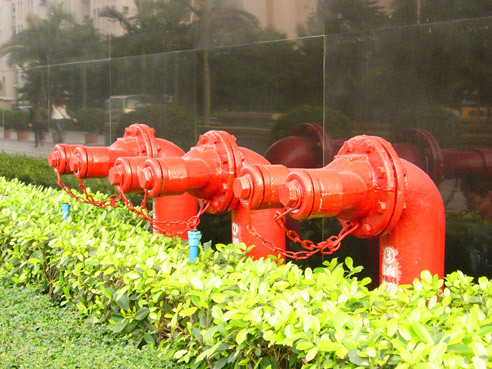This outdoor photograph captures a scene brimming with contrast and vibrant colors, focusing on three bright red industrial fire hydrants situated in front of a large, reflective building. The building is covered in shiny black tiles sectioned by silver lines, resembling large squares. In the reflective tiles, one can see a mirrored image of the surroundings, including elements such as palm trees, a car, and people walking nearby.

Nestled against the base of the building is a low, bright green hedge, which extends across the foreground and contrasts sharply with the red hydrants. The hydrants, designed for emergency use, feature two nozzle connections each, secured by red chains to prevent loss of the caps. Near the bottom left corner of the image, there is a patch of green grass adding to the color composition.

Further details include two blue pipes emerging from the green bush in front of the hydrants, likely part of the landscaping irrigation system. In the background, mixed in with the mirrored reflections on the building’s surface, one can see a blend of trees and other natural elements, harmonizing the urban and natural aspects of the scene.